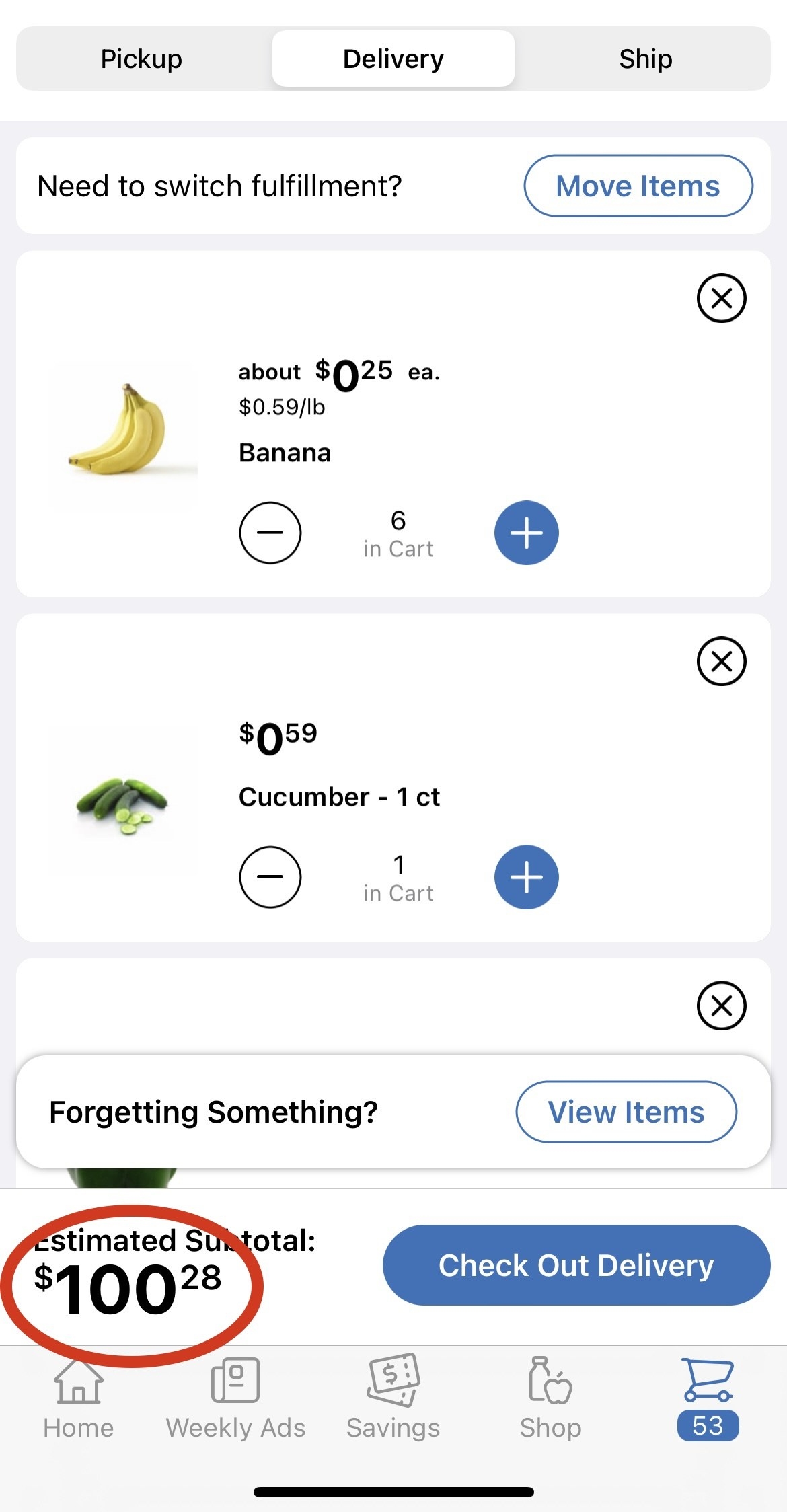This is a comprehensive vertical rectangular image portraying an interactive shopping interface design.

**Top Section:**

- **Background:** Solid gray.
- **Text Elements:**
  - "Pickup" in bold black font, placed at the top left.
  - Central element: A horizontal white box with "Delivery" in bold black letters.
  - "Ship" in black font, back on the gray background.

**Middle Section:**

- **Outline:** Light gray or light blue horizontal line creating divisions.
- **Interactive Area:**
  - Upper top edge features a prompt, "Need to switch fulfillment?" in black font. 
  - Adjacent to it, a clickable element: "Move items" in blue font placed inside a white oval with a blue outline.

**Product Listing Section:**

- **First Item:**
  - **Image:** Banana icon on the left.
  - **Price Information:**
    - Line 1: About $0.25 ea.
    - Line 2: $0.59 per lb.
    - Line 3: "Banana" in bold font.
  - **Cart Section:**
    - Minus symbol inside a white circle with a black rim.
    - "In Cart" in light gray with the number 6 above.
    - Plus symbol in a blue circle.

- **Second Item:**
  - **Image:** Cucumber icon on the left.
  - **Price Information:**
    - $0.59
    - "Cucumber - 1 ct" in lowercase.
  - **Cart Section:**
    - Minus symbol inside a white circle with a black rim.
    - "In Cart" with the number 1 above.
    - Plus symbol in a blue circle.

**Additional Prompts and Information:**

- **Reminder Section:**
  - Prompt: "Forgetting something?" in bold black font.
  - Interactive button: "View items" in blue font within a white oval with a blue outline.
  - Black 'X' symbol inside a circle for closure on the top right corner.

- **Subtotal Information:**
  - "Estimated subtotal: $100.28" in bold black font.
  - Entire subtotal is encircled with a bold red oval.
  - Adjacent interactive oval: "Checkout delivery" in white text within a blue oval.

**Bottom Navigation Section:**

- **Links with Icons:**
  - "Home," "Weekly Ads," "Savings," and "Shop" from left to right, each with corresponding icons.
  - Final element: Blue shopping cart icon with a small blue oval, "53" in white text.
- **Footer:** A thick, bold black line centered at the very bottom.

This image offers a comprehensive interface mock-up highlighting various interactive shopping options and relevant product details.